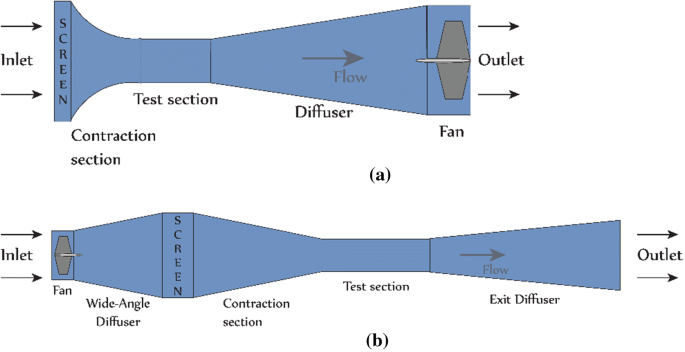The image showcases two designs of mini wind tunnels, labeled A and B, each delineated with a series of components and directional flows. 

In design A, depicted in blue, the wind tunnel begins with an inlet, followed by a screen. The flow then progresses through a contraction section into a test section. After the test section, the airflow moves into a diffuser, then passes a fan, and finally exits through an outlet marked by two arrows pointing to the right.

Design B, situated below the first, starts with an inlet and two black arrows pointing to the right. It features a fan, which feeds into a wide-angle diffuser that contains a screen. The airflow then continues through a contraction section and a test section. From the test section, the air moves through an exit diffuser, marked by a right-pointing arrow labeled "flow," and finally exits through an outlet indicated by two arrows pointing to the right. The images and components are clearly labeled to elucidate the stages of airflow through each wind tunnel.